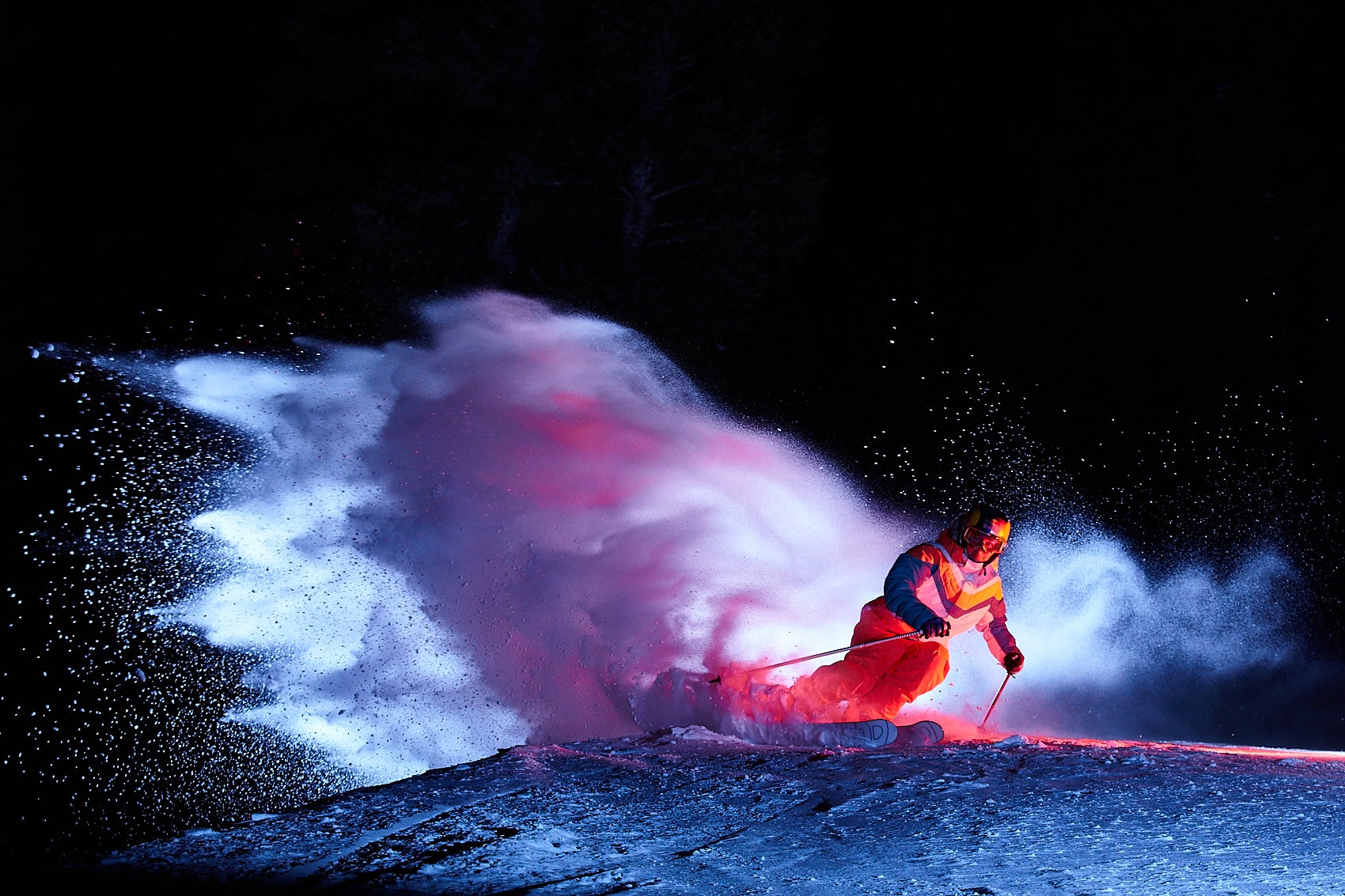In this striking nighttime photograph, a skier is captured mid-action, carving a sharp turn and sending a spectacular plume of powdery snow into the air. The scene is dramatically lit by a spotlight, which casts a lavender hue on the snowy mist and an orange glow on the skier's legs. The skier, possibly male, is clad in a vibrant outfit featuring orange ski pants, a blue helmet adorned with orange and yellow, and a multi-colored ski jacket with shades of blue, white, and orange. He is equipped with ski poles in both hands, the left one planted in the snow while the right one hovers in the air, adding to the dynamic composition. Against the pitch-black sky, the airborne ice crystals appear as tiny white specks, their motion frozen by a fast shutter speed, creating a dynamic illusion of being suspended in time. The skier's pink goggles and the intense focus in their gaze add to the heightened atmosphere of what seems to be an advertisement, showcasing the exhilarating essence of night skiing.